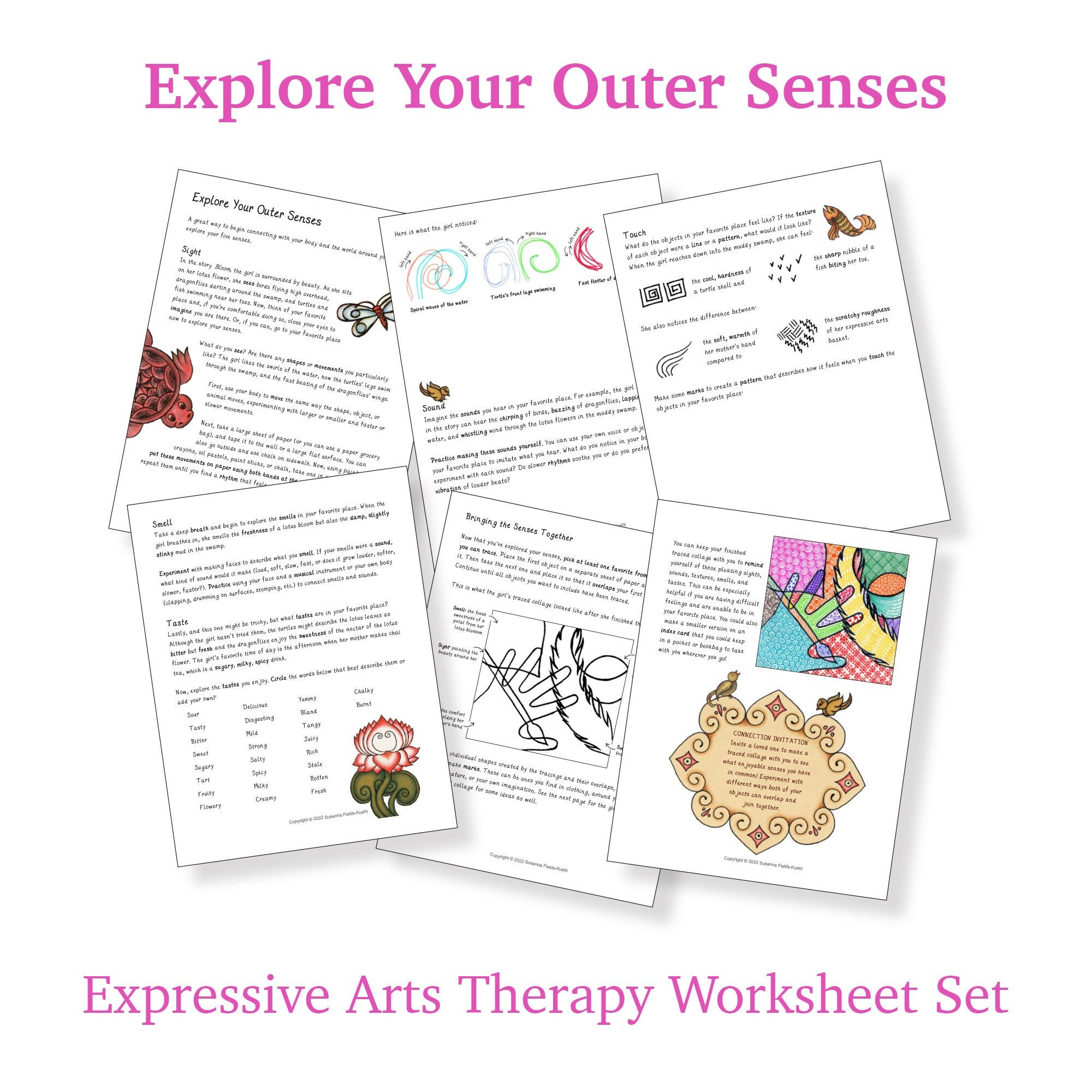This image features an advertisement for an "Expressive Arts Therapy Worksheet Set," framed with a white background. At the very top in a purple font, it says "Explore Your Outer Senses," and at the bottom, it reads "Expressive Arts Therapy Worksheet Set." Six worksheets are showcased in two horizontal rows of three. The worksheets are small, white vertical rectangles with black text that is difficult to read due to its size. 

The top left worksheet at an angle shows illustrations of a turtle and a butterfly. The top middle worksheet, which angles to the left, includes several circles, though their purpose is unclear. The top right worksheet, also angled to the left, features a fish and other symbols in black and white.

In the bottom row, the bottom left worksheet, angled to the left, displays a flower illustration. The bottom middle worksheet, angled to the right, depicts a hand touching a feather. The bottom right worksheet, similar in content to the one next to it but colored in various clashing hues, also angles to the right. Despite the small text, these worksheets seem designed for engaging in different artistic and sensory activities.